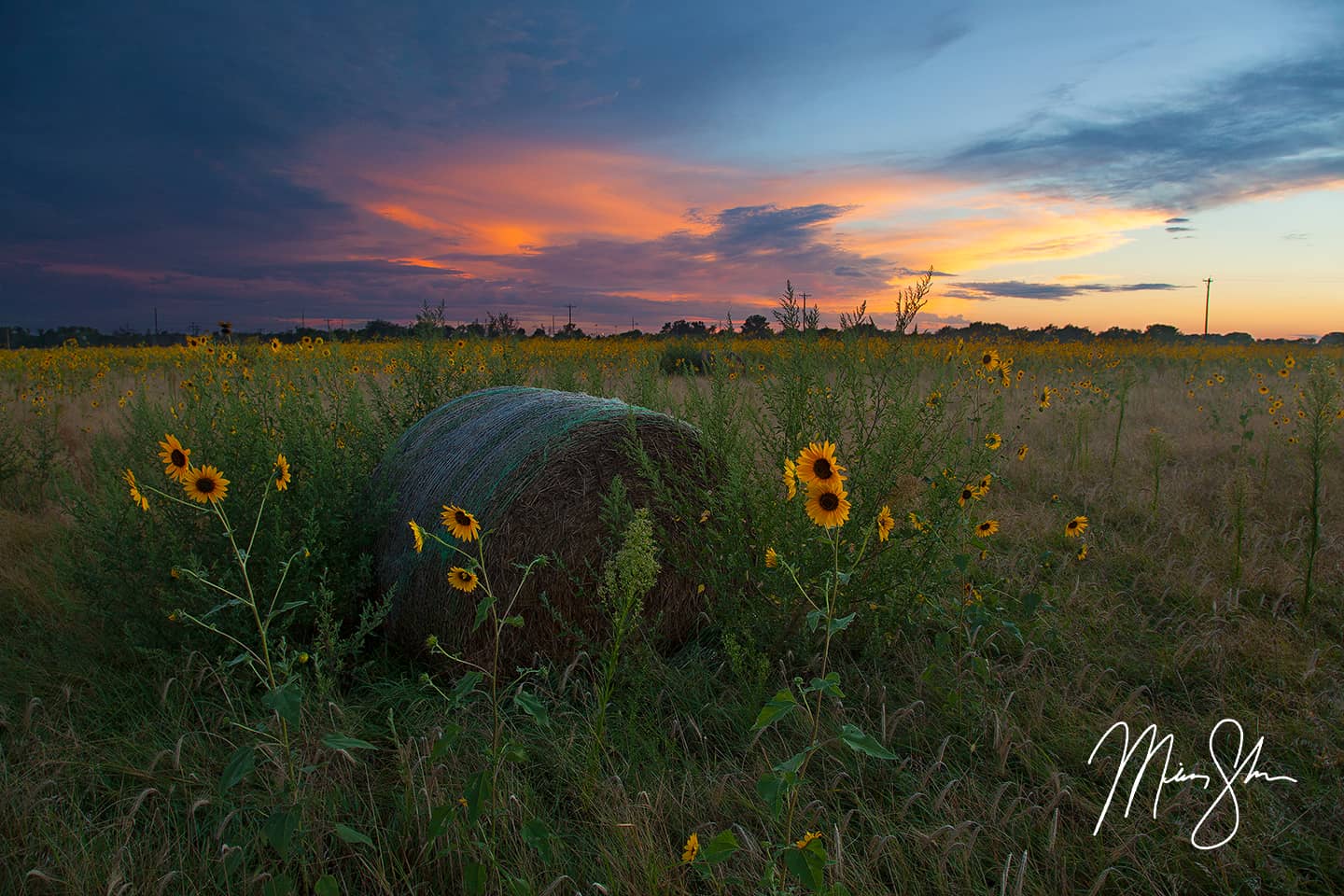This outdoor photograph captures a serene field scene at sunset or sunrise, distinguished by a signature in white at the bottom right corner, with the initials M and S, although the full name is not legible. The sky is a striking tapestry of orange, gray, and darker blue clouds with a hint of light blue at the top. Below the vibrant sky, a line of leafy trees frames the horizon. The foreground features a lush grassy field dotted with tall sunflowers or similar yellow flowers with brown centers. Dominating the center, slightly left of the middle of the image, is a large, perfectly round bale of hay. The composition balances various elements of nature, creating a picturesque countryside landscape.